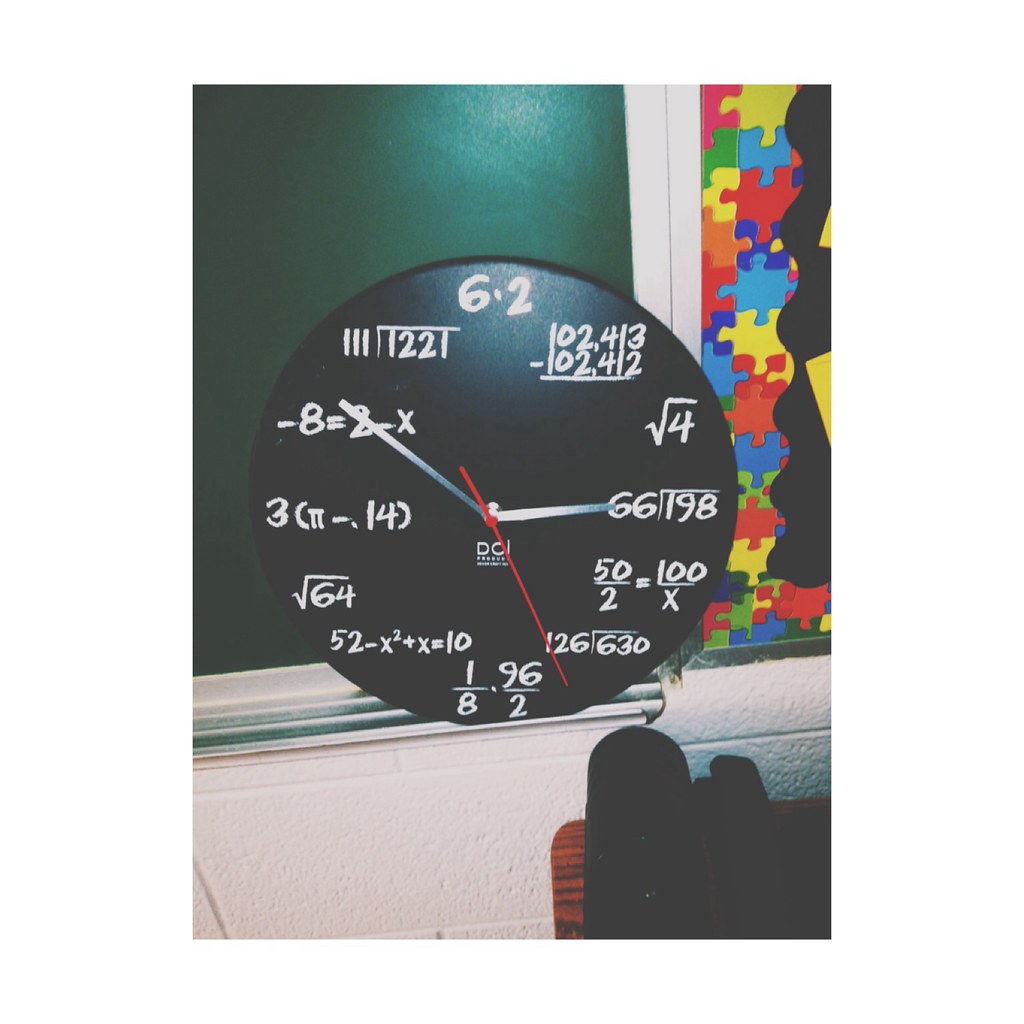The photograph captures a unique clock resting against a green chalkboard, with the bottom of the clock settled on the chalkboard’s metal rail. The clock features a silver hour hand, minute hand, and a red second hand, with the time set to approximately 10:27. Instead of numerals, the clock face displays twelve mathematical expressions in white chalk-style writing. For example, at 12 o'clock, it reads "6 times 2", at 1 o'clock, "102.413 minus 102.412", and at 2 o'clock, "the square root of 4". The black circular clock contrasts sharply with the chalkboard. Adjacent to the chalkboard, a colorful bulletin board adorned with a jigsaw puzzle piece print and black lines is visible. The room's background includes parts of a white cinder block wall and a brown table with a few black objects on it. The entire scene evokes an academic atmosphere, blending mathematical whimsy with traditional classroom elements.